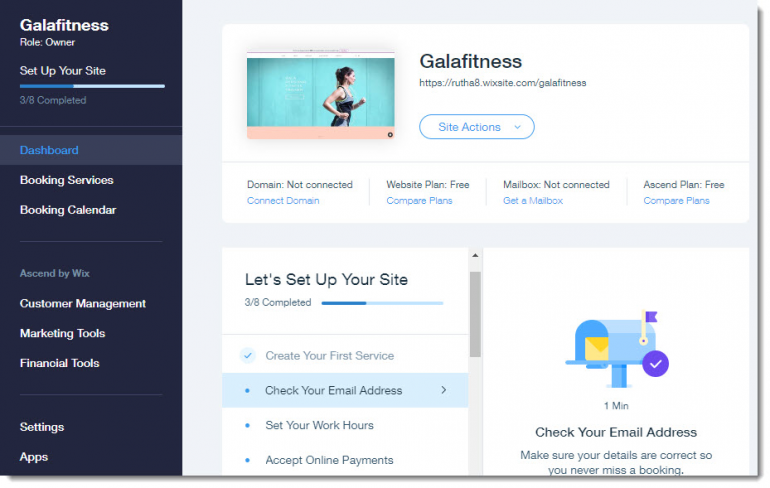This screenshot from Gala Fitness displays a comprehensive setup interface for managing the fitness service platform. 

On the left sidebar, there's an elongated blue bar indicating the navigation menu, featuring sections such as "Gala Fitness," "Role Owner," and "Set Up Your Site." The progress indicator shows that 3 out of 8 setup steps are complete. The sidebar items include "Dashboard," "Booking Services," "Booking Calendar," with the "Dashboard" highlighted in blue as the selected option. Additional sections noted are "Ascend by Wix," "Customer Management," "Marketing Tools," "Financial Tools," "Settings," and "Apps."

The central part of the image features a clean white background with an image of a woman running, dressed in a blue workout outfit. The branding "Gala Fitness" is prominently displayed, followed by a URL link under it: ruthate.wixsite.com/galafitness.

Below the link, there is a white button with blue text labeled "Site Actions," accompanied by a downward arrow. Beneath it, there are notifications for "Domain not connected" with an option to connect the domain, "Website Plan (Free)" with a prompt to compare plans, and “Mailbox not connected” with an option to get a mailbox. The text also notes "Ascend Plan (Free)" and provides options to compare plans.

A progress box underlines the setup status, displaying "Let's Set Up Your Site" with 3 out of 8 steps completed. A progress bar visualizes this status. Tasks for site completion are listed: "Create your first service" (checked), "Check your email address" (arrow pointing right), "Set your work hours," and "Accept online payments." An image of a mailbox with a purple checkmark and the text "1 minute" is noted beneath, emphasizing the importance of verifying email details to ensure no bookings are missed. The right side features a scrollbar for additional navigation within the setup interface.

Overall, the caption captures the detailed interface layout of Gala Fitness's setup page, highlighting its structured design and essential setup tasks.